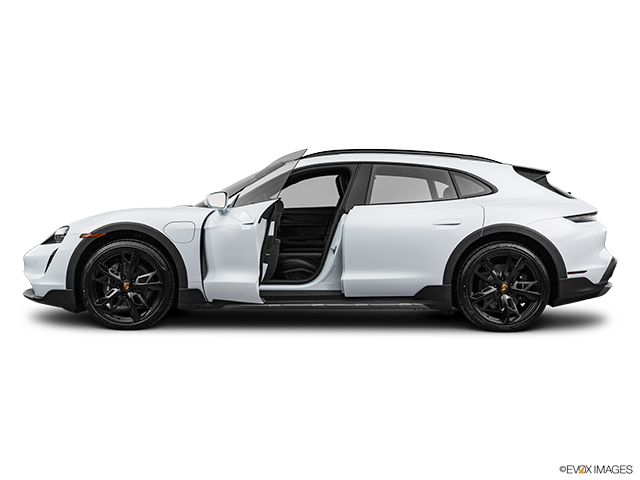This is a photograph of a white electric vehicle, likely an SUV, taken from the driver's side profile with its front facing towards the left and its rear towards the right. The image has a rectangular shape, with the top and bottom sides being twice as long as the left and right sides, and features a solid white background and surface. The vehicle has a sleek, sloped roof towards the rear, which is more pronounced due to its elongated hood. It has four doors, with the front driver's side door open, revealing a black interior. The vehicle is equipped with black rubber tires with five-spoke black rims. The car's windows are tinted gray, and there is a black sunroof on top. In the bottom right corner of the photograph, there is a "EVOX Images" watermark, reinforcing that the car is an electric vehicle.